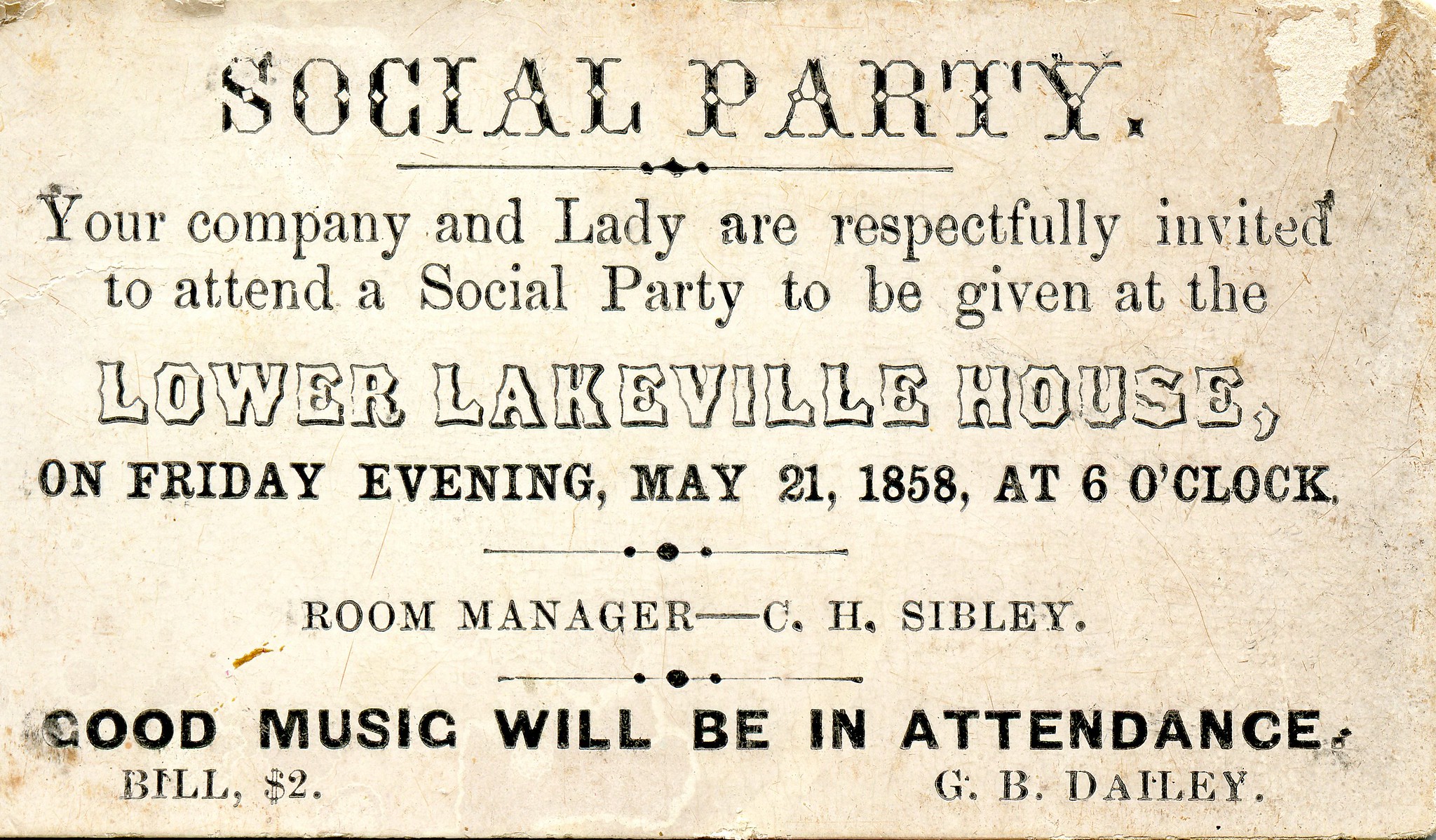The image is a photograph of a weathered and discolored invitation from the 1800s, likely for an old-fashioned event. The frayed edges and worn paper indicate its age. At the top, in bold, black letters, it reads "Social Party" with a horizontal black line beneath it. The main body of the text states: "Your company and lady are respectfully invited to attend a social party to be given at the Lower Lakeville House on Friday evening, May 21, 1858 at 6 o'clock." Below this, another line separates the details. It lists the room manager as C.H. Sibley and emphasizes, in bold letters, that "Good music will be in attendance." Additionally, on the bottom left corner, the bill is noted as $2, and on the bottom right, the name G.B. Daily is printed. This is clearly an invitation to a social event from 1858, highlighting music and managed by C.H. Sibley.